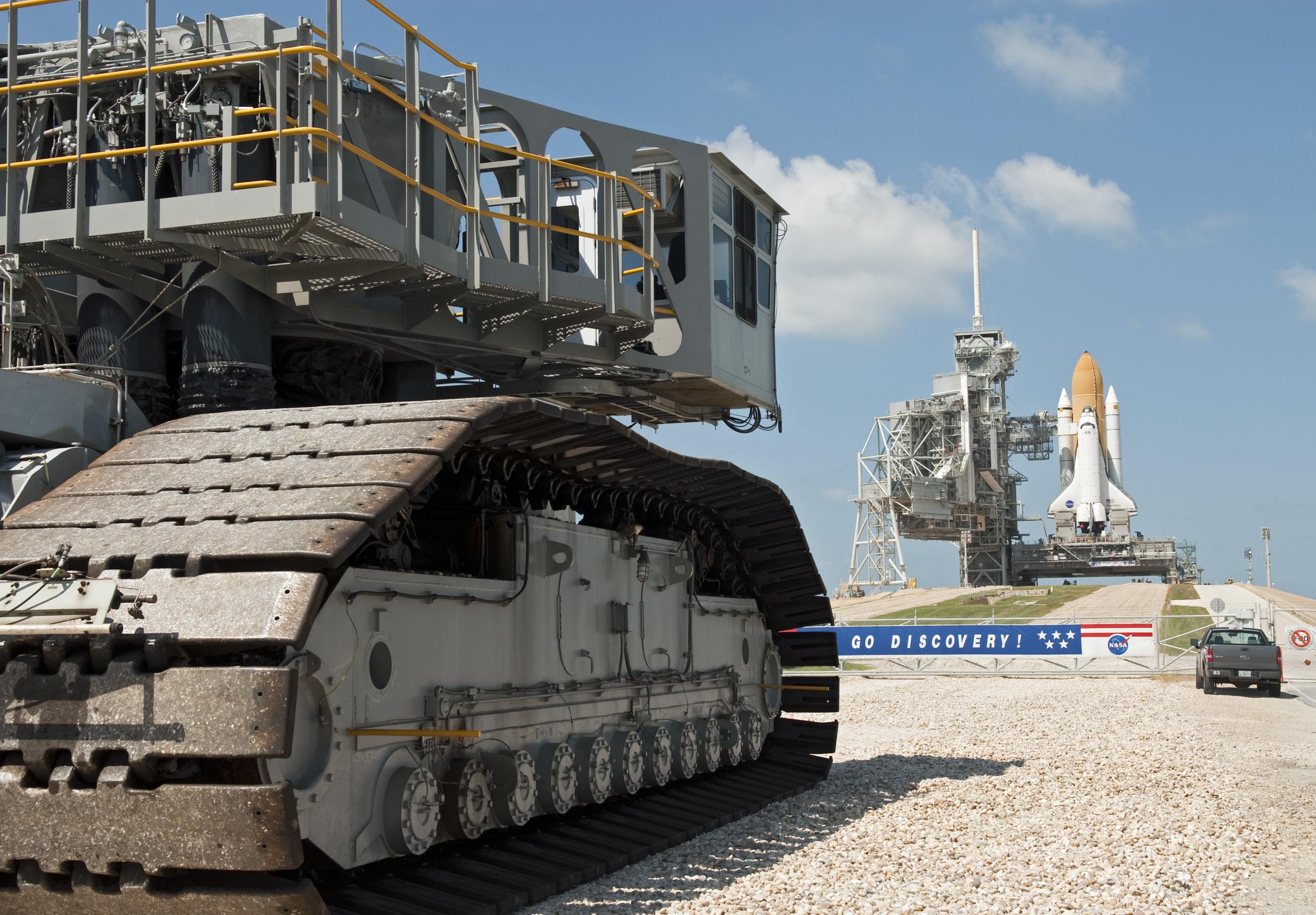The image is a clear, bright, and sunny day at a NASA launch site featuring a rocket on the launchpad, ready for takeoff. A prominent banner reading "Go Discovery!" with the NASA logo and five stars is displayed, adding to the anticipatory atmosphere. In front of a fence marking off the launch area, a dark grey truck is parked, emphasizing the restricted zone. The foreground showcases a unique command vehicle resembling a tank, equipped with all-terrain, caterpillar tracks typical of heavy construction machinery, possibly used to flatten the ground or transport other equipment. The sky is a vivid blue with scattered cirrus clouds, and the ground is covered with gravel and rocks, highlighting the rugged environment essential for such high-stakes operations. The scene is devoid of people, focusing on the impressive technology and machinery orchestrating the upcoming space launch.